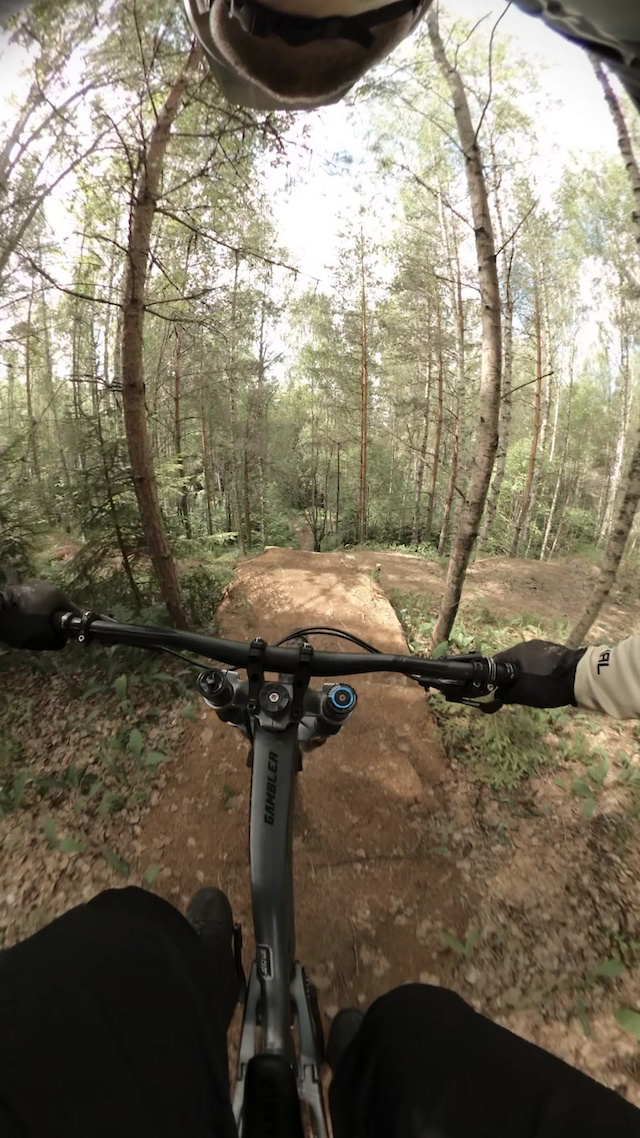In this photograph, captured with a chest-mounted action camera, likely a GoPro, we see the perspective of a cyclist riding a black bike through forested dirt trails. The image has a fisheye lens effect, creating a distorted, bubble-like appearance. Framed with the cyclist's knees at the bottom and the chin just at the top, we can see their black gloves gripping the black handlebars.

The cyclist is clad in black pants, black shoes, and a tan long-sleeved shirt. The trail ahead appears reasonably straight, lined with sparse, thin-trunked trees that are beginning to lose their leaves, suggesting it might be fall. The forest ground on either side of the pathway is littered with leaf matter. The sky above is clear but glaringly bright, with patches of blue visible through the canopy. The sunlight illuminates the scene, contributing to the overall clarity and atmosphere of the photograph.